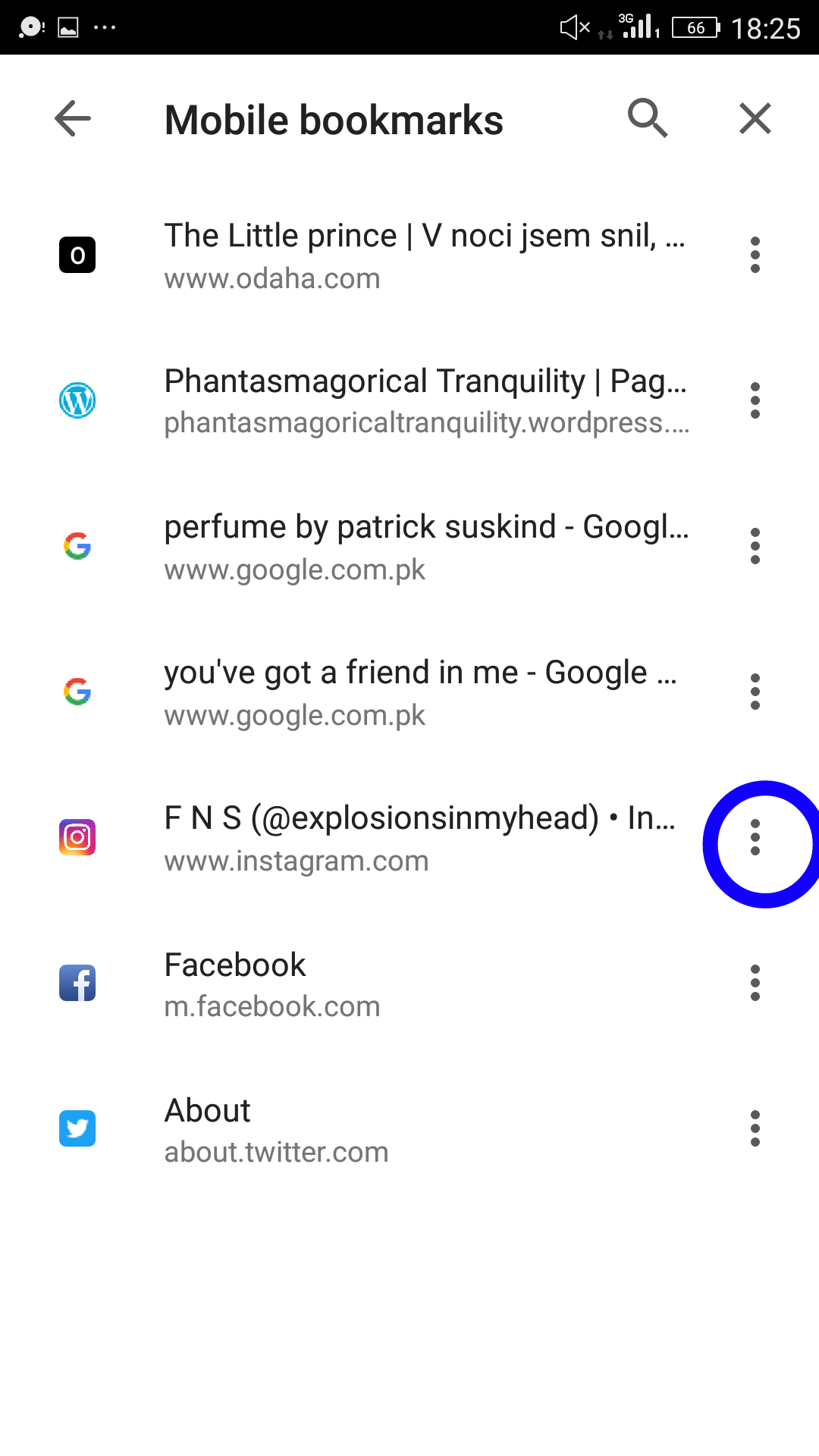Screenshot of an Android phone displaying the "Mobile Bookmarks" page. The bookmarks listed are as follows:

1. **"The Little Prince"** - Pointing to the website www.odaha.com.
2. **"Phantasmagorical Tranquility"** - Appears to be a blog hosted on phantasmagoricaltranquility.wordpress.com.
3. **"Perfume by Patrick Suskind"** - Links to a Google address.
4. **"You've Got a Friend in Me"** - Another bookmark linking to a Google search.
5. **"FNS (at explosions in my head)"** - Points to an Instagram page.
6. **"Facebook"** - The mobile version of Facebook.
7. **"About"** - The Twitter About page.

The interface of the Android device is clearly visible, showing the organization and title of each bookmark.